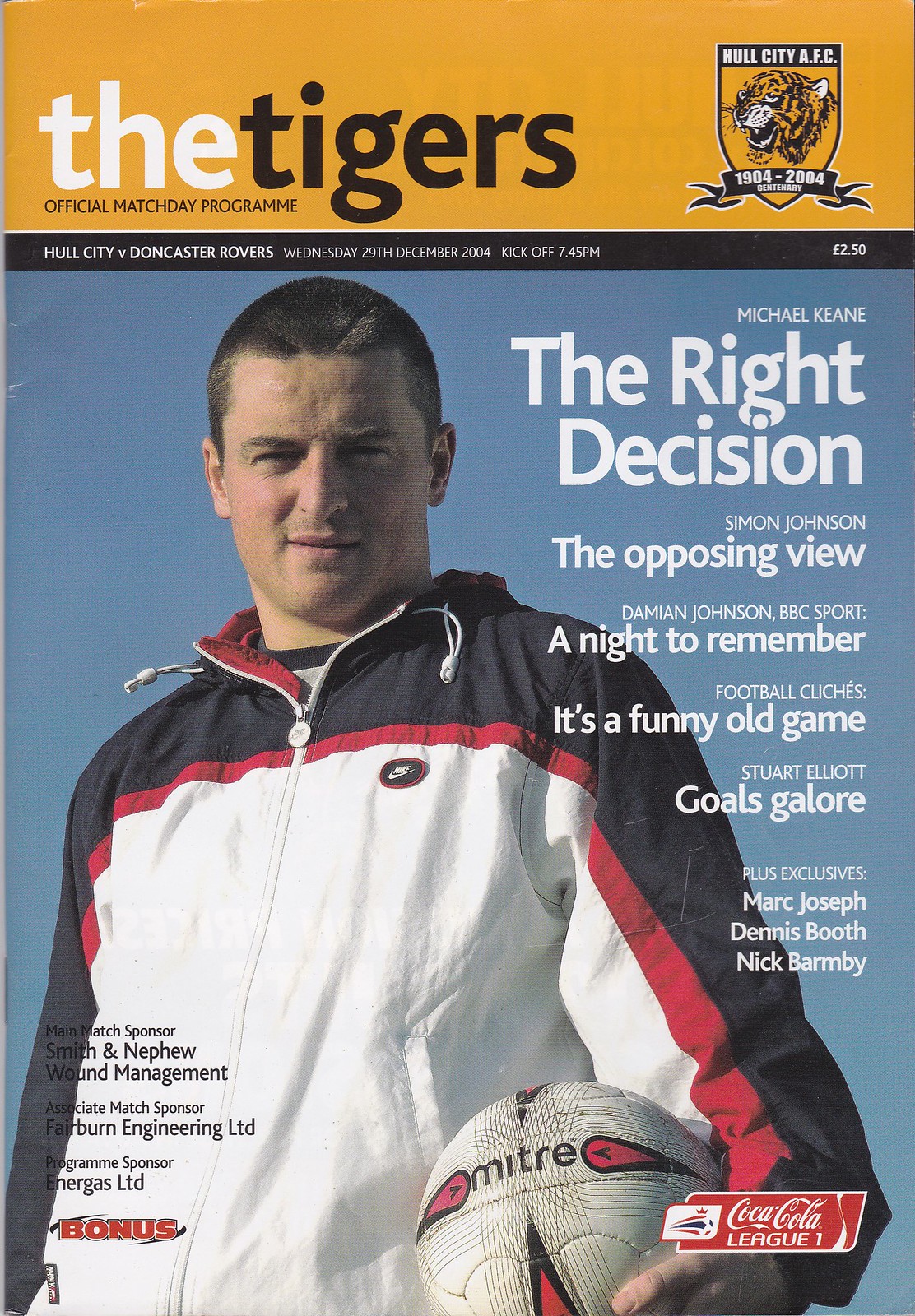The magazine cover, rectangular in shape with dimensions about six inches tall by four inches wide, features an identifiable design and specific details. The top quarter has an orange background with a yellow strip. On the left, in bold white and black lowercase letters, it reads "the Tigers." Beside this, a shield-shaped logo displays "Hull City A.F.C." with a tiger image and the dates 1904-2004.

Beneath the orange area, a thin black stripe stretches across the width, adorned with white lettering stating, "Official Match Day Program: Hull City vs. Doncaster Rovers, Wednesday 29th December 2004, kickoff 7:45 p.m. £2.50." 

The image's primary focus below this header is a man of Caucasian descent, sporting a very short crew cut, and looking directly at the viewer. He is dressed in a distinctive windbreaker jacket—white at the bottom, with a red stripe above it, and black on the upper sections near the shoulders and sleeves. In his left hand, he holds a white Mitre soccer ball with red accents.

To the right of the man, in white text, the magazine features several headings: "Michael Keane: The Right Decision," "Simon Johnson: The Opposing View," "Damian Johnson, BBC Sport: A Night to Remember," "Football Clichés: It's a Funny Old Game," "Stuart Elliott: Goals Galore," and "Plus Exclusives: Mark Joseph, Dennis Booth, Nick Barmby." 

Additional details include black font at the lower left for sponsors: "Main Match Sponsor: Smith and Nephew Wound Management," "Associate Match Sponsor: Fairburn Engineering LTD," and "Program Sponsor: Energis LTD," with "Bonus" written in red print. The bottom right corner features a red advertisement for "Coca-Cola League One."